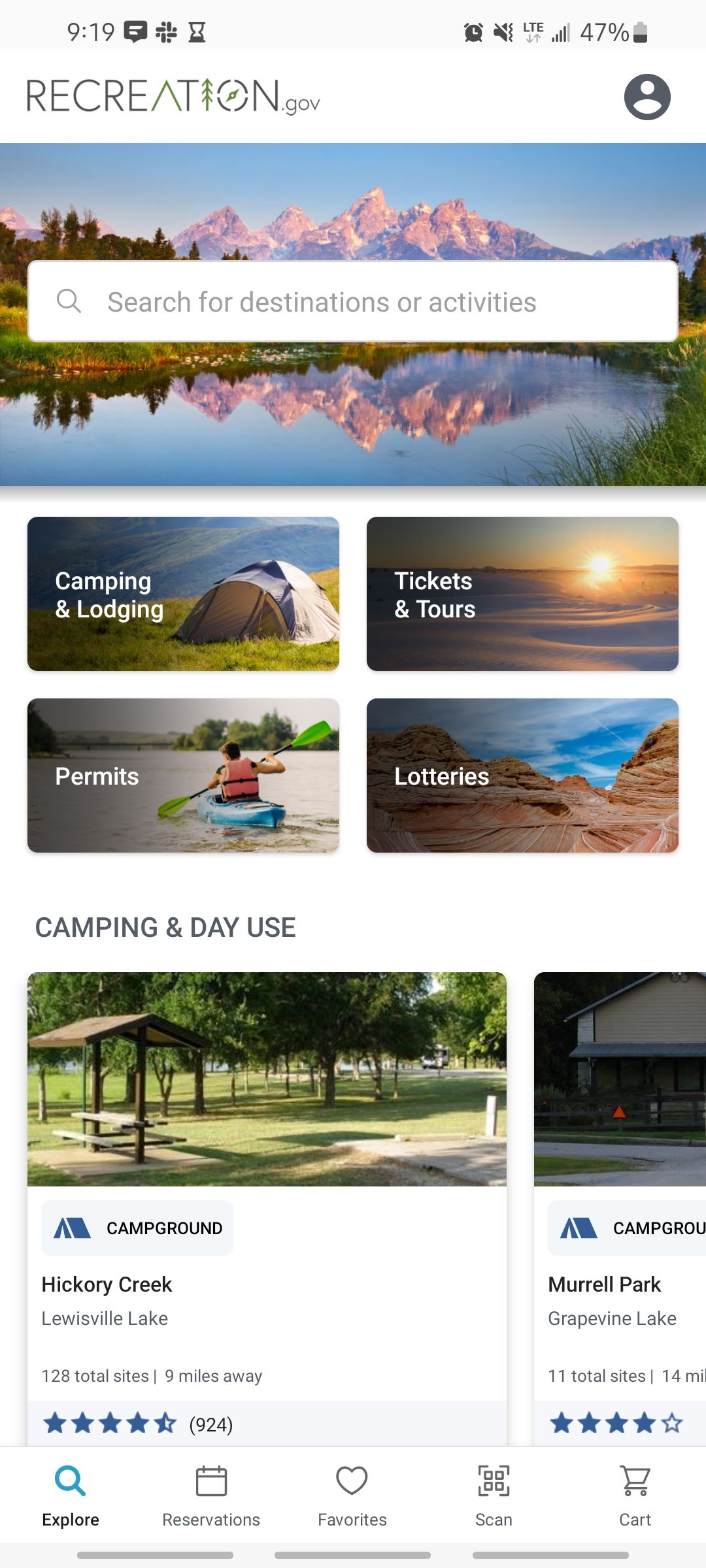A picturesque scene showcases a recreational area managed by recreation.gov. In the foreground, a modern LTE speaker with 47% battery sits prominently. The backdrop is a stunning landscape with majestic mountains under a brilliant blue sky, lush green trees, and a pristine body of water framed by rectangular shapes. The area features various outdoor facilities including campgrounds, lodges, and tent sites, all surrounded by verdant grass. On offer are tickets and tours for sun-soaked adventures on sandy shores, and permits are available for kayaking, complete with oars and kayaks. Camping and day-use spots are detailed, with Hickory Creek Campground at Lewisville Lake 9 miles away, spanning 120 acres, rated 4.5 stars by 924 visitors. Memorial Park near Grapevine Lake is also mentioned, noted for its variety. Additional details include a reference to a "lunch list" featuring amenities like Blue Men, fine glass objects, reservations, and assorted favors. Below the image, a sequence of three gray lines adds a subtle design element.